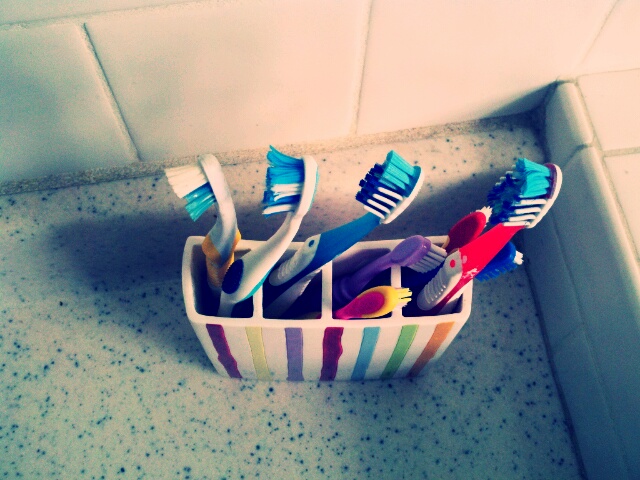This top-down, bird's-eye view photograph captures a white, multi-colored striped toothbrush holder, segmented into four slots, each filled with toothbrushes. The stripes on the holder include dark purple, green, lighter purple, blue, and orange. In the first slot on the left, there are three toothbrushes: a white and yellow one, a white and blue one, and a yellow-bristled toothbrush. The second slot contains a blue and white toothbrush. The third slot holds two smaller children's toothbrushes, one red and yellow and the other purple. The fourth slot on the right houses two tall red and white toothbrushes with blue bristles. The holder sits on a granite surface with blue speckles, and nearby white tiled walls are visible, providing a clean, organized bathroom setting.